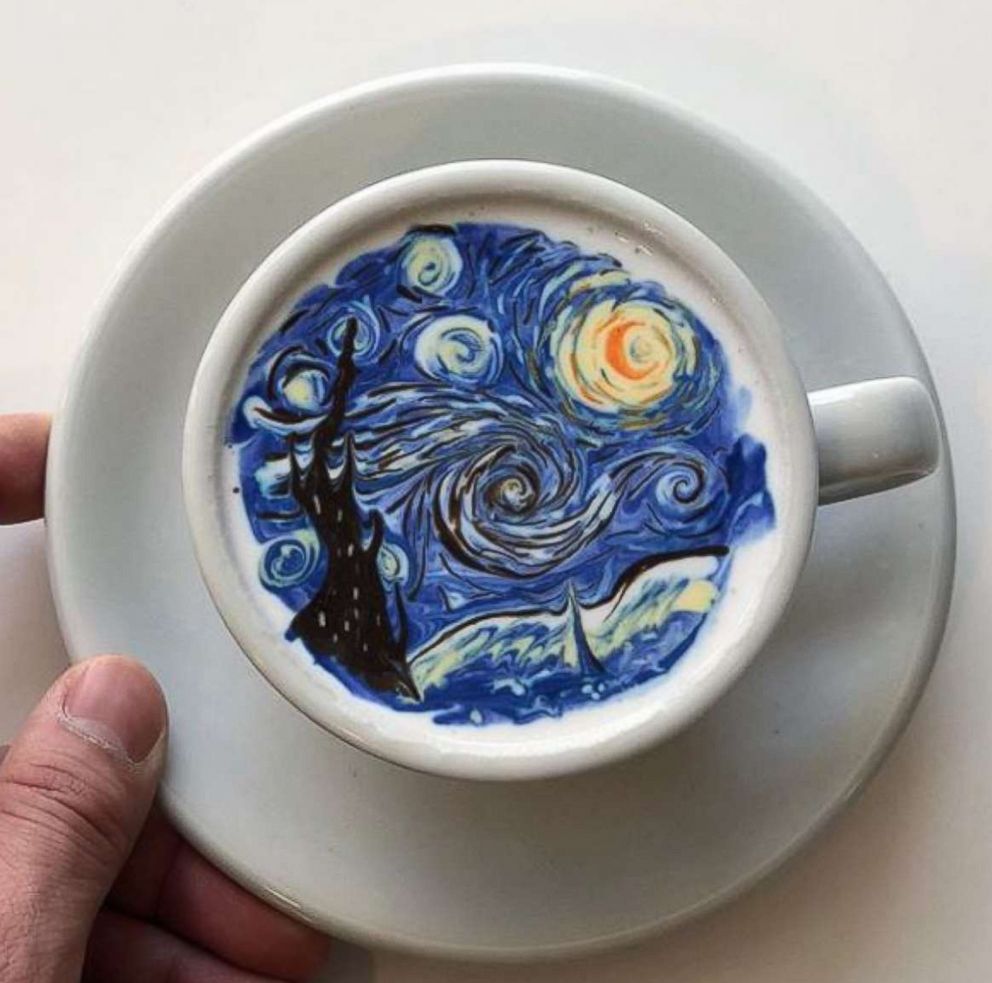This square photograph, captured from a top-down perspective, showcases an intricately crafted latte art within a white coffee cup centered on a matching white saucer. The handle of the cup is positioned to the right side of the image, while the bottom left corner reveals a Caucasian person's thumb and fingers gently touching the saucer. The background remains stark white, emphasizing the focal point—the coffee's surface adorned with an exquisite replication of Vincent van Gogh's "Starry Night." This detailed foam art displays the iconic swirls of blue, black, yellow, and orange, closely mirroring the famous painting's blend of colors and abstract patterns. The remarkable precision of the artwork within the small cup transforms the ordinary coffee experience into a visual masterpiece.